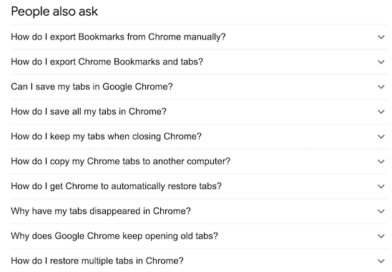Displayed in the image is a partial page of search engine results. The content appears to address a series of queries related to managing bookmarks and tabs in Google Chrome. The primary heading reads, "People also ask," followed by a list of expandable questions that remain unopened. These questions include: 

- "How do I export bookmarks from Chrome manually?"
- "How do I export Chrome bookmarks and tabs?"
- "Can I save my tabs in Google Chrome?"
- "How do I save all of my tabs in Chrome?"
- "How do I keep my tabs when closing Chrome?"
- "How do I copy my Chrome tabs to another computer?"
- "How do I get Chrome to automatically restore tabs?"
- "Why have my tabs disappeared in Chrome?"
- "Why does Google Chrome keep opening old tabs?"
- "How do I restore multiple tabs in Chrome?"

The context suggests that the original search query pertained to managing Chrome bookmarks and tabs, which is further evidenced by the related questions listed. This resource could be particularly beneficial for Chromebook users who may be unfamiliar with these features, offering potential solutions and guidance directly related to their queries. However, in the image, all questions remain in a collapsed state, presenting the user with options but no immediate answers.